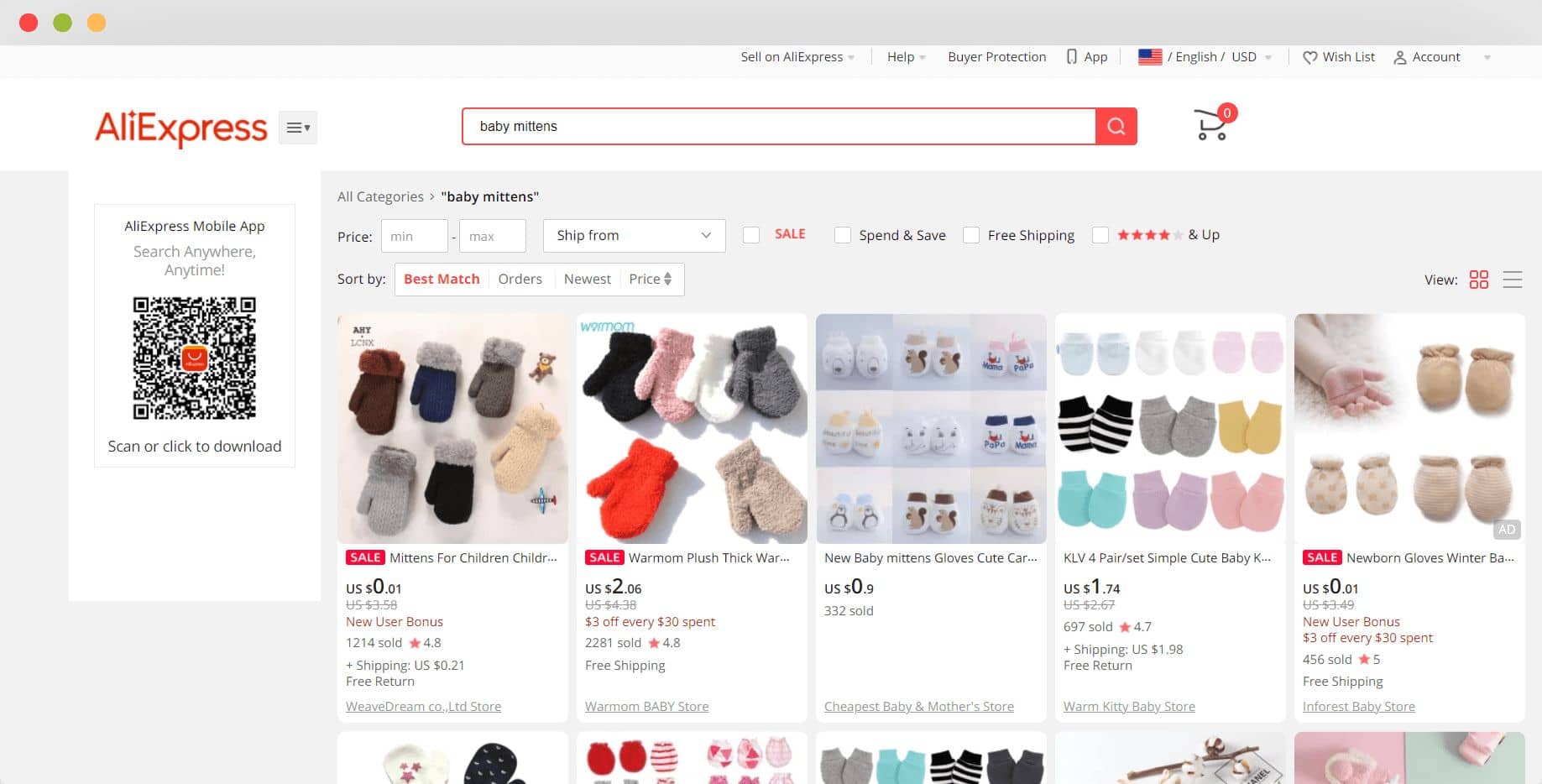The image depicts a screenshot of someone using the AliExpress mobile app. In the top left corner, there are three colored circles: the first one is red, the second green, and the third yellow. On the right-hand side, there are options labeled "Sell on AliExpress," "Help," and "Buy a Protection App." Below these, an American flag icon beside text indicating English and USD is visible, followed by heart and account icons for wishlist and user profile respectively.

The background colors are predominantly white and red, with "AliExpress" prominently displayed on the left-hand side. A white search box with a red border is centered, with the query "baby mittens" typed in. To the right of the search box is a black shopping cart icon with a red circle at the top indicating zero items.

On the bottom left, there is a QR code with an AliExpress shopping bag design beneath it, accompanied by the text "Scan or click to download." Above this, a caption reads "AliExpress mobile app, search anywhere, anytime."

The main content shows a list of search results for baby mittens. Each item includes a thumbnail and details such as:
1. Mittens for children - priced at $0.01 for new users.
2. Warm mom plush thick mittens - priced at $2.06, with a promotion of $3 off every $30 spent.
3. New baby mittens gloves - priced at $0.90, with 332 units sold.
4. Simple cute baby mittens by KLV - priced at $1.74, with 797 units sold.

The prices are displayed in U.S. dollars, with new user bonuses and discounts highlighted in red.